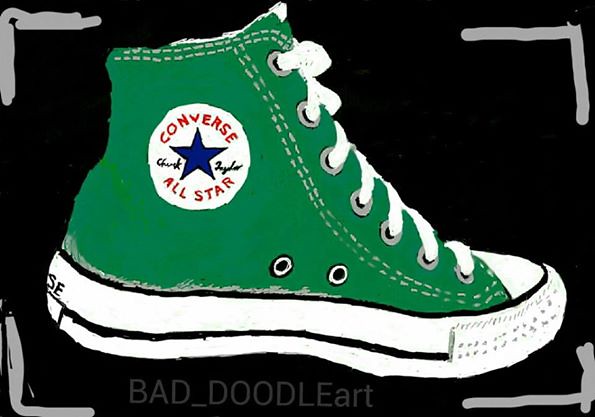The image is a detailed sketch of a green Converse high top sneaker against a predominantly black background. Each corner of the background features a loose, right-angle line in light gray, reminiscent of a camera viewfinder. The sneaker is depicted in a sideways view and is laced up with white laces. The tongue and front of the shoe are also white, with silver-tone grommets for the laces. The sole is white, topped with a black horizontal line through its center and additional black lines on the lower sole. On the side of the shoe, near the ankle, there is the iconic circular Converse logo, comprising red text that reads "CONVERSE" and "ALL STAR," a blue star in the center, and the cursive script "Chuck Taylor" in black. Additionally, two vent holes are visible near the shoe’s base. At the bottom of the image, there is a caption that reads "BAD_DOODLE_ART" in uppercase gray text. The back of the shoe displays the letters "S-E," suggesting more text that is partially obscured.